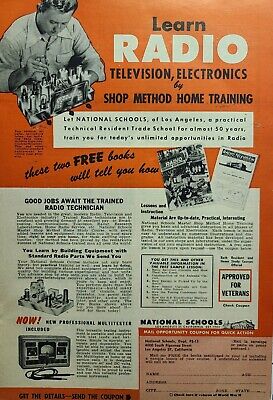The image is an old magazine advertisement from the 1940s or 1950s, characterized by an orange background. At the top, it prominently displays the phrase "LEARN RADIO TELEVISION ELECTRONICS BY SHOP METHOD HOME TRAINING." Below, it features a paragraph that reads: "Let National Schools of Los Angeles, a practical technical resident trade school for almost 50 years, train you for today's unlimited opportunities in radio." 

The advertisement includes a black-and-white picture of a young man in the upper left-hand corner, dressed in a white button-down collared long-sleeved shirt, working on what appears to be an old-style radio. Additional smaller images of various electronic devices and radios are also present.

Towards the bottom, the text mentions "These two free books will tell you how" and "Good jobs await the trained radio technician," emphasizing the prospects of employment. It further explains, "You learn by building equipment with standard radio parts we send you." There is a section in the bottom right-hand corner for readers to fill in their name and address to request more information, although the smaller text is difficult to read.

The overall tone and style of the advertisement reflect its vintage nature, invoking a nostalgic appeal to historical home-training methods for aspiring radio technicians.